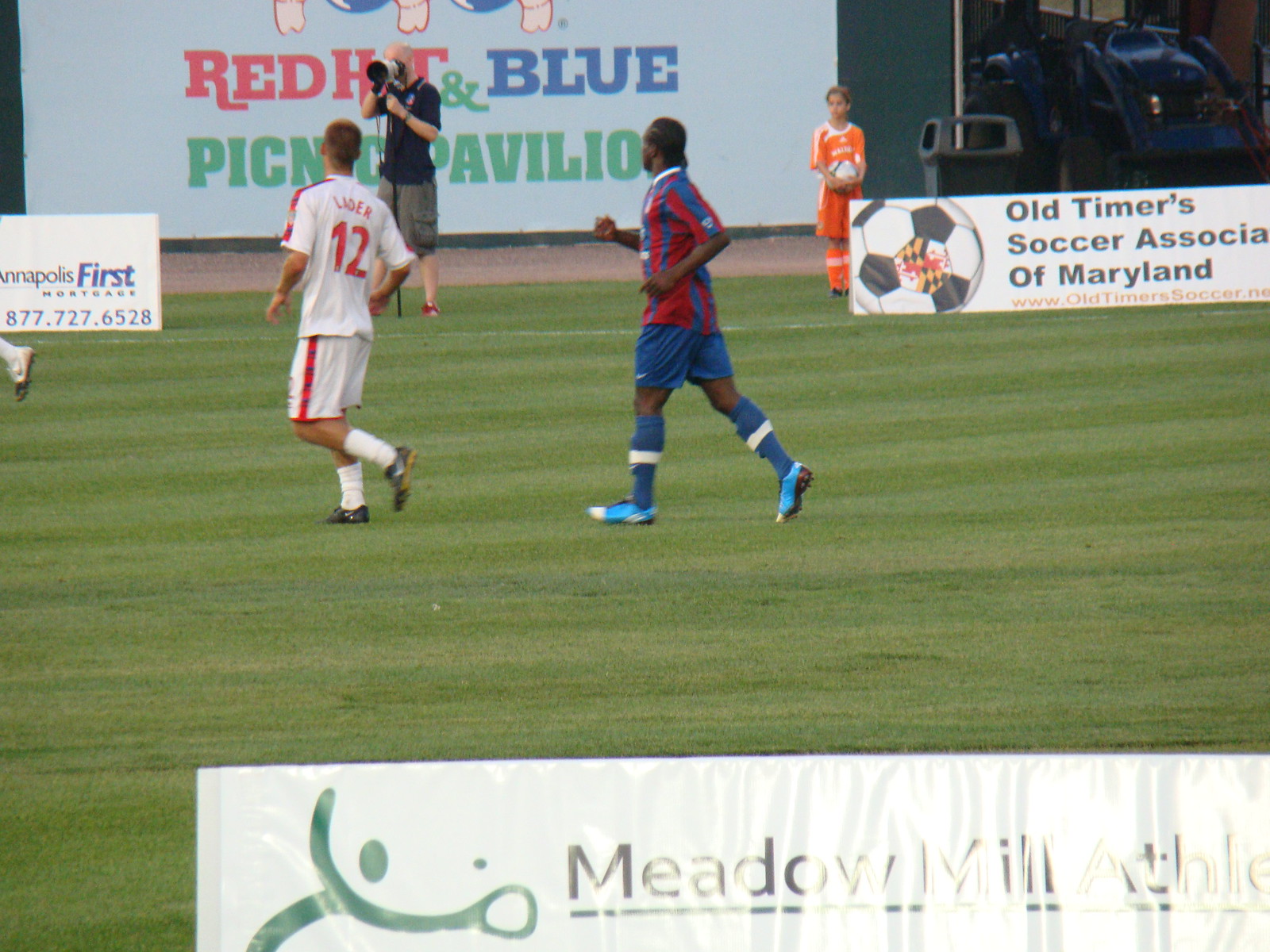This photograph captures a vivid outdoor, daylight soccer scene featuring two players at the focal point on a lush green soccer field. One player, identifiable as Litter by his jersey, is wearing a white uniform accented with red stripes and bearing the number 12. Adjacent to him is another player with dark skin, donning a blue and red uniform. Behind them, a man in a black polo shirt and khaki shorts holds a large camera, ready to capture the action. Over to the right, a young child, dressed entirely in orange, holds a soccer ball. The background reveals various signs and banners: prominently, a large sign for "Red Hot and Blue Picnic Pavilion" with "Red" and "Hot" in red text, "Blue" in blue text, and "Picnic Pavilion" in dark green. Another visible sign advertises the "Kannapolis First Mortgage" with the phone number 877-727-6528. Additionally, there's a banner for the "Old-Timer Soccer Association of Maryland" featuring a soccer ball and their website, www.oldtimersoccer.net. The scene is bustling with activity, encapsulated by the dynamic surroundings and the detailed elements captured in this lively photograph.